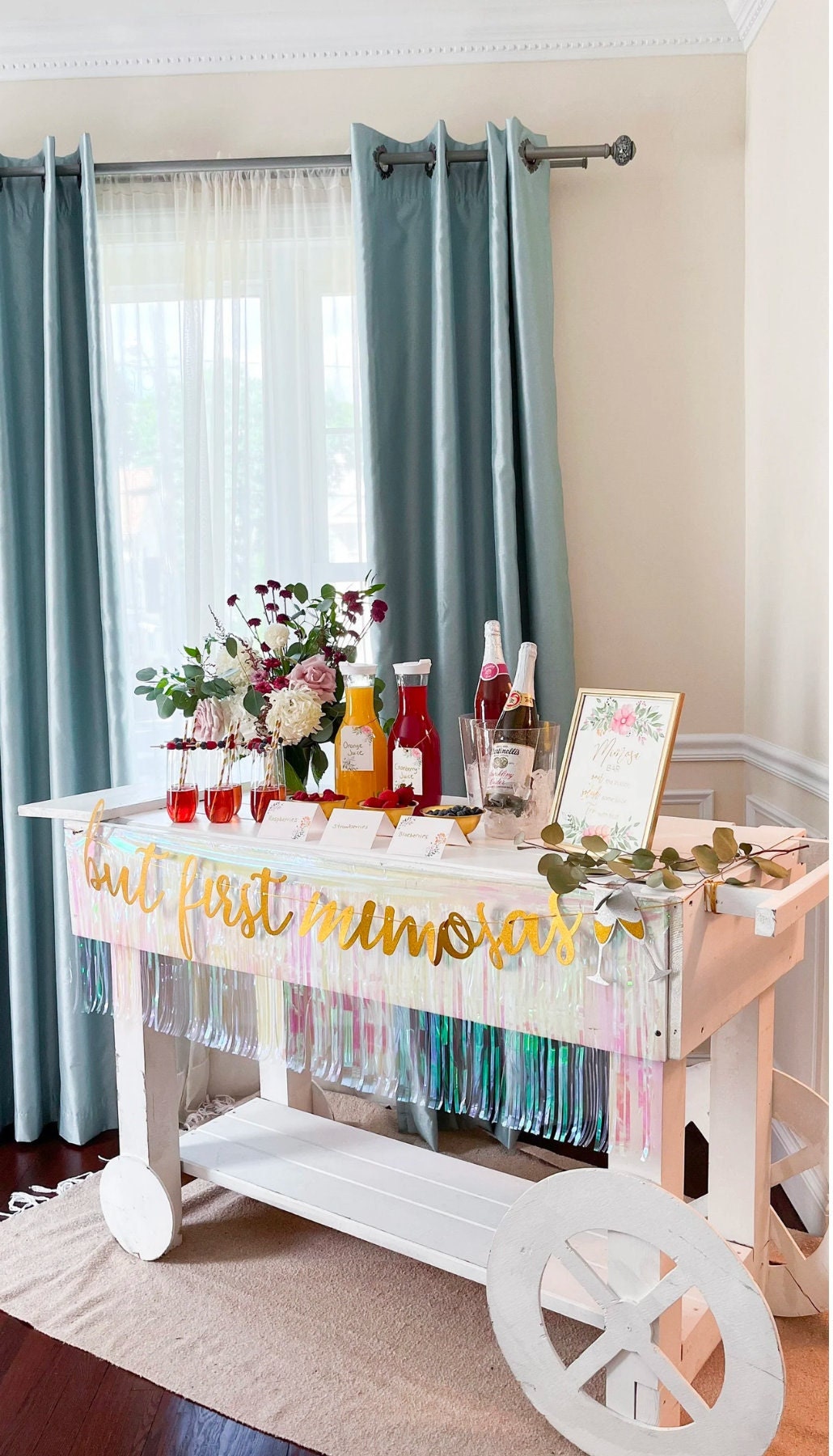The photograph captures a small wooden decorative cart, painted entirely in white, designed to display drinks or foods. The cart features two large flat white-painted wheels at the back and two smaller white-painted wheels at the front. It resembles a table, with three white planks at the bottom connecting the four legs, and a box-like counter structure on top. The cart has a wooden handle on one side of the counter. Covering the top of the cart is a metallic, see-through tablecloth. 

Across the front of the cart, there is a gold text banner that reads, "But First Mimosas," with an illustration of two clinking wine glasses. On the top of the cart, there are three red glasses, each half-filled with a red liquid, decorated with mixed berries on the rims and straws inside. A vase with a floral arrangement containing pink, white, and red roses adds a decorative touch. The cart also holds pitchers of orange juice and cranberry juice, several bottles including some that appear to be Martinelli’s sparkling cider, ketchup, and mustard, as well as small glass buckets possibly containing champagne. 

The cart is situated in a room with a light-colored rug over a wood floor. It is positioned slightly to the left in the image, near the corner where a light-colored wall meets gray or green curtains hanging by a window. Some delicate white curtains are also visible closer to the window. The overall setting gives a charming and celebratory feel.